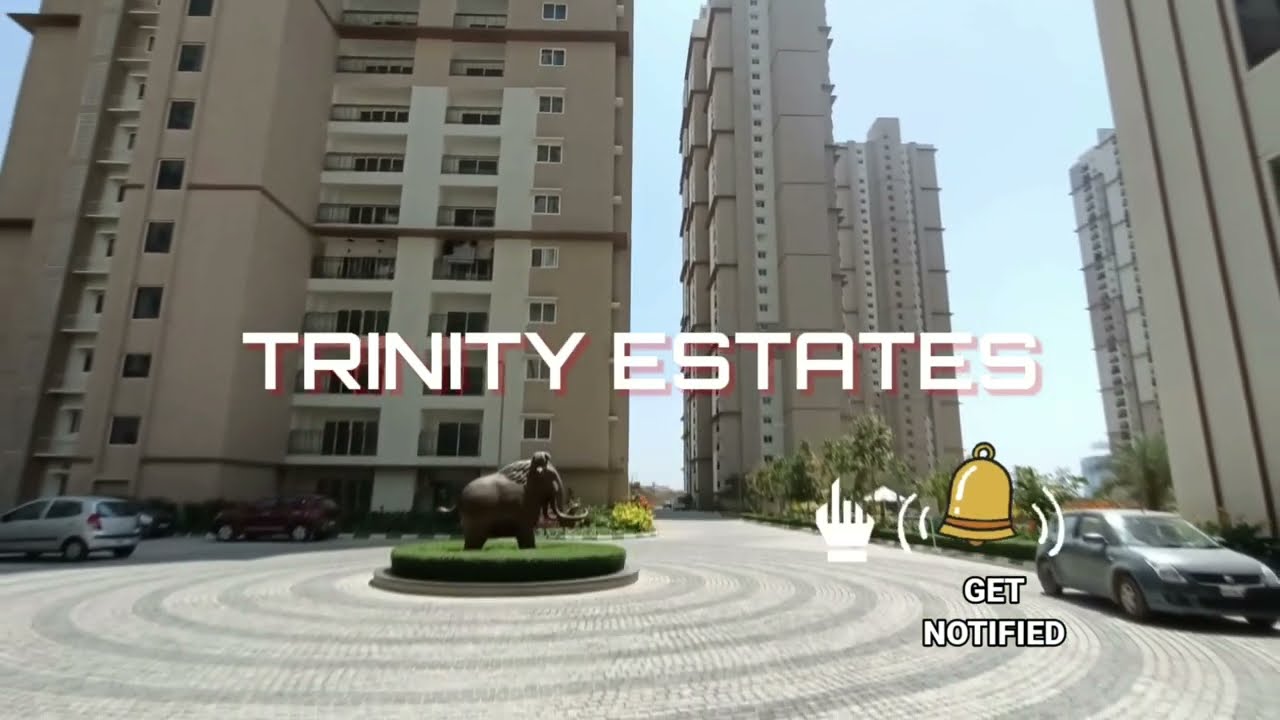The image likely depicts a frame from a commercial or possibly a promotional sign for a company or property named "Trinity Estates." In the center, the text "Trinity Estates" is prominently displayed in white, capital letters with a red shadow effect. Just below the text, there is a yellow bell symbol with curved lines indicating sound waves and adjacent white text that reads "Get Notified."

The background features a meticulously maintained circular grassy area, with a bronze-colored statue of an elephant situated centrally. This statue is surrounded by neatly arranged concentric rings of gray and white stones.

To the bottom right of the image, there's a light gray hatchback vehicle. On the left, two more vehicles, one gray and one tan, are parked near the tall apartment buildings. These buildings, beige in color, are several stories high adorned with balconies and numerous windows, with some balcony levels framed in white.

The primary colors dominating the scene are light blue and tan, giving the overall composition a clean and inviting atmosphere.